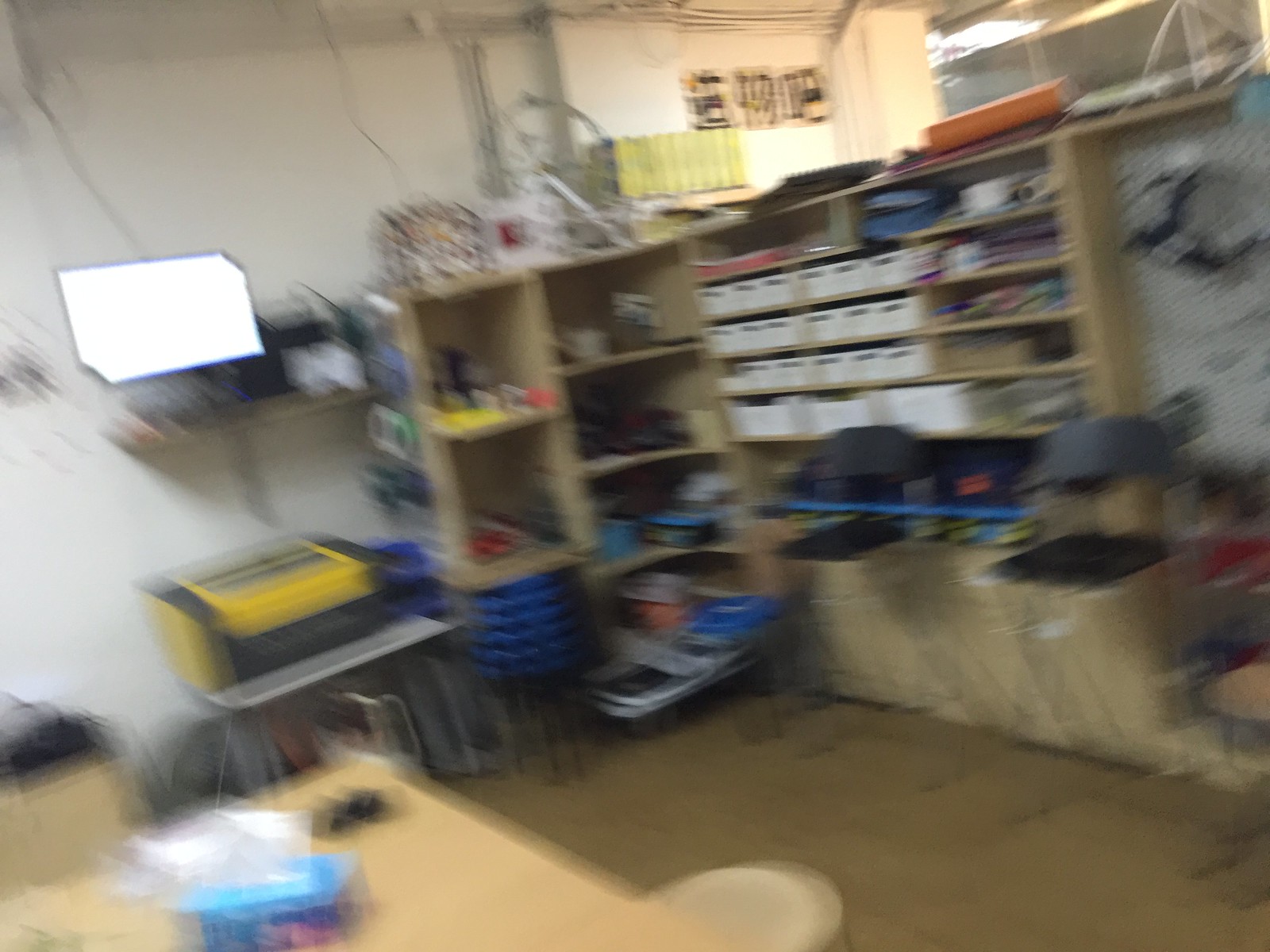This photograph, though out of focus due to motion, captures the interior of a building with white walls. On the right-hand side, multiple shelves are lined with white bins. In front of these shelves, there are a couple of black-seated chairs. A desk is partially visible in the bottom left-hand corner, adorned with a blue Kleenex box. The back wall features a computer monitor perched on a shelf, and below it, on a grey desk, sits a yellow and black machine. A room divider is situated behind the shelves, revealing a brightly lit adjacent room on the other side.